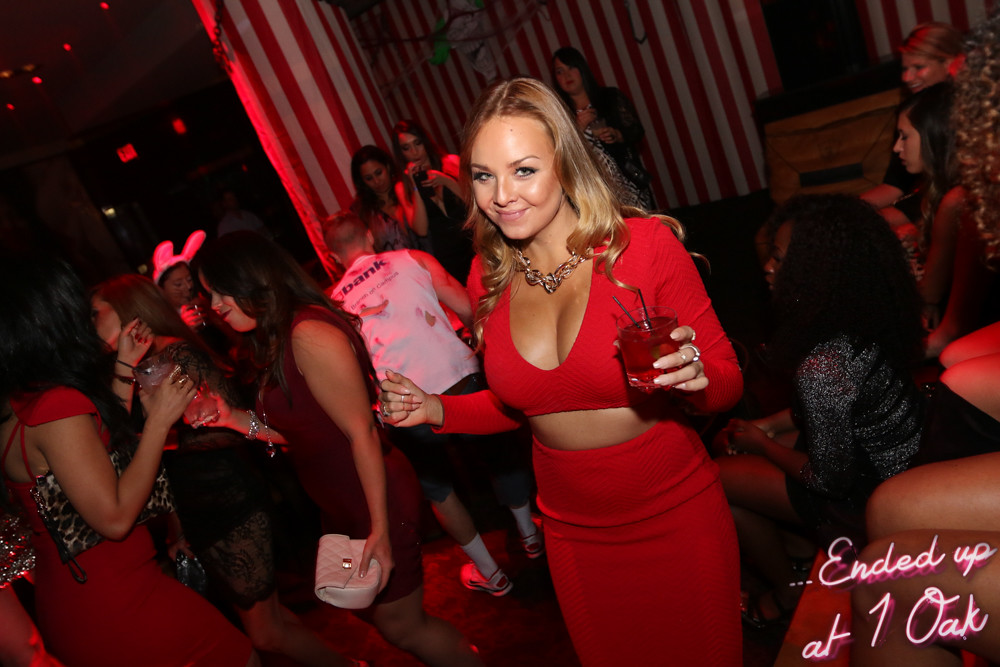The photograph captures a vibrant scene at a nightclub or dance party, likely at a venue called One Oak, as suggested by the caption styled in a handwritten, neon sign-inspired font in the lower right corner: "...ended up at one oak." 

In the foreground, a young, attractive Caucasian woman with long, blonde hair that cascades over her shoulders is the centerpiece. Her hair is parted in the middle, slightly pulled away from her face, with the ends curled. She is dressed in an eye-catching, low-cut red dress with long sleeves and a bare midriff, revealing a bit of her decolletage. The dress contours her figure, elegantly showcasing her curves. Complementing her look, she wears a chunky gold necklace adorned with what appear to be rubies.

The woman's cheerful smile is directed straight at the camera, exuding a sense of enjoyment and confidence. She holds a red cocktail with two straws in her left hand, positioned towards the right side of the image, while her right hand suggests she might be dancing. Her pose and the setting give the impression that she is actively engaged in the night’s festivities.

The background features a dimly lit dance floor with red lighting and silhouettes of other attendees, most of whom are dressed in red, white, or black—possibly hinting at a Valentine's Day event or mixer. To her left, people appear to be dancing, while to the right, others can be seen seated in the shadows, adding depth to the lively atmosphere. This detailed and dynamic image could easily be used in promotional material or social media to highlight the energetic nightlife scene at One Oak.